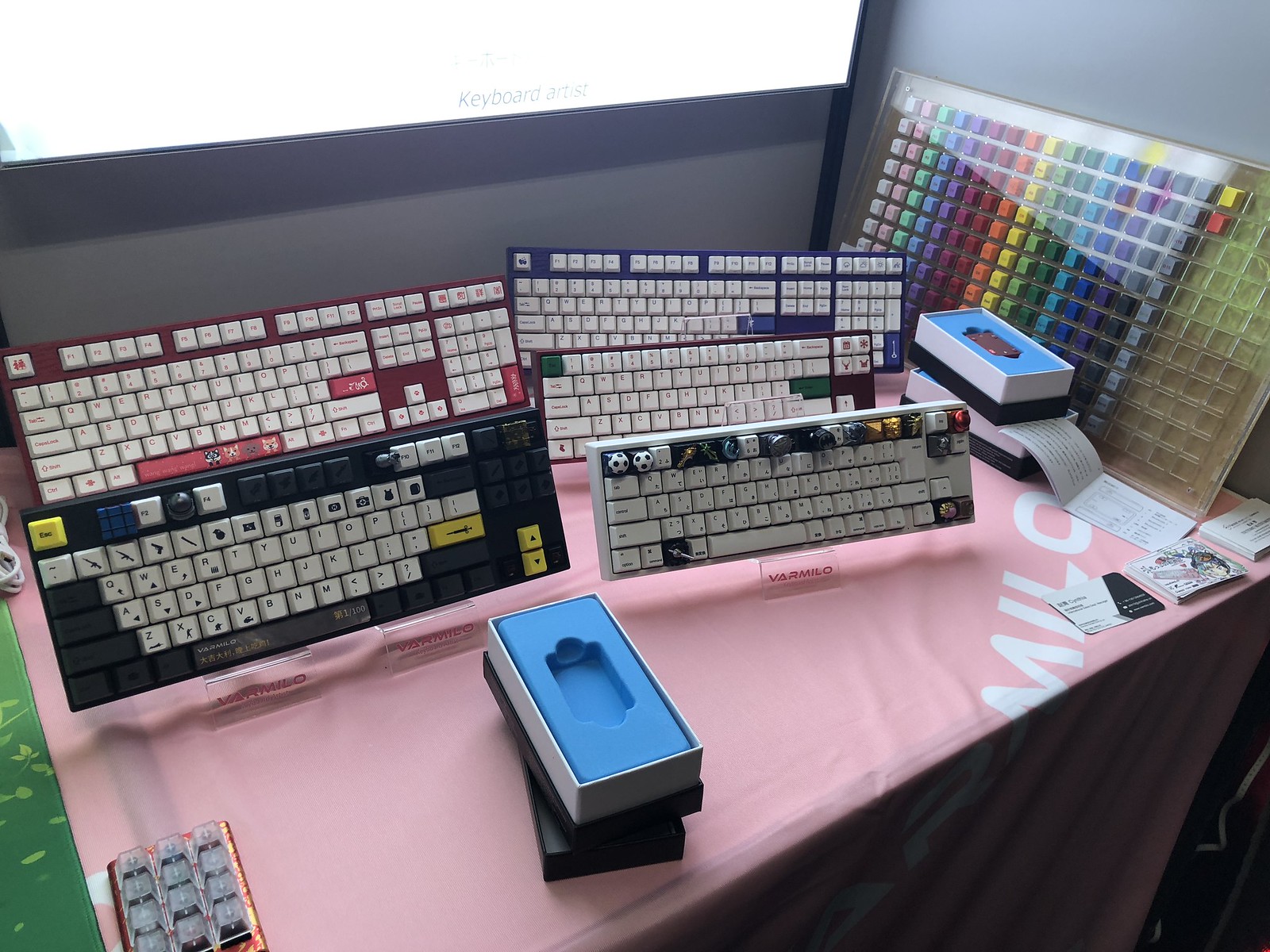In the image, there is a gray wall resembling a TV or projector screen in the background. Positioned against this wall is a yellow table covered with a pink tablecloth. Arranged neatly on this table are five different computer keyboards, displayed upright. The keyboards are of varying colors: purple, red, black, blue, and white, with most of their keys being white. Some of the keys on the top row of two keyboards feature unique symbols such as soccer balls, a chess piece, and dice. Alongside the keyboards are several black, white, and blue boxes, which appear to be open and empty. The tablecloth has the letters "M-I-L-O" visible on it. Additionally, there are several business cards scattered on the table. A glass or plastic container holding various colorful keyboard buttons sits in one corner of the table. Lastly, a device with numerous colorful buttons is mounted on the wall to the right of the display.